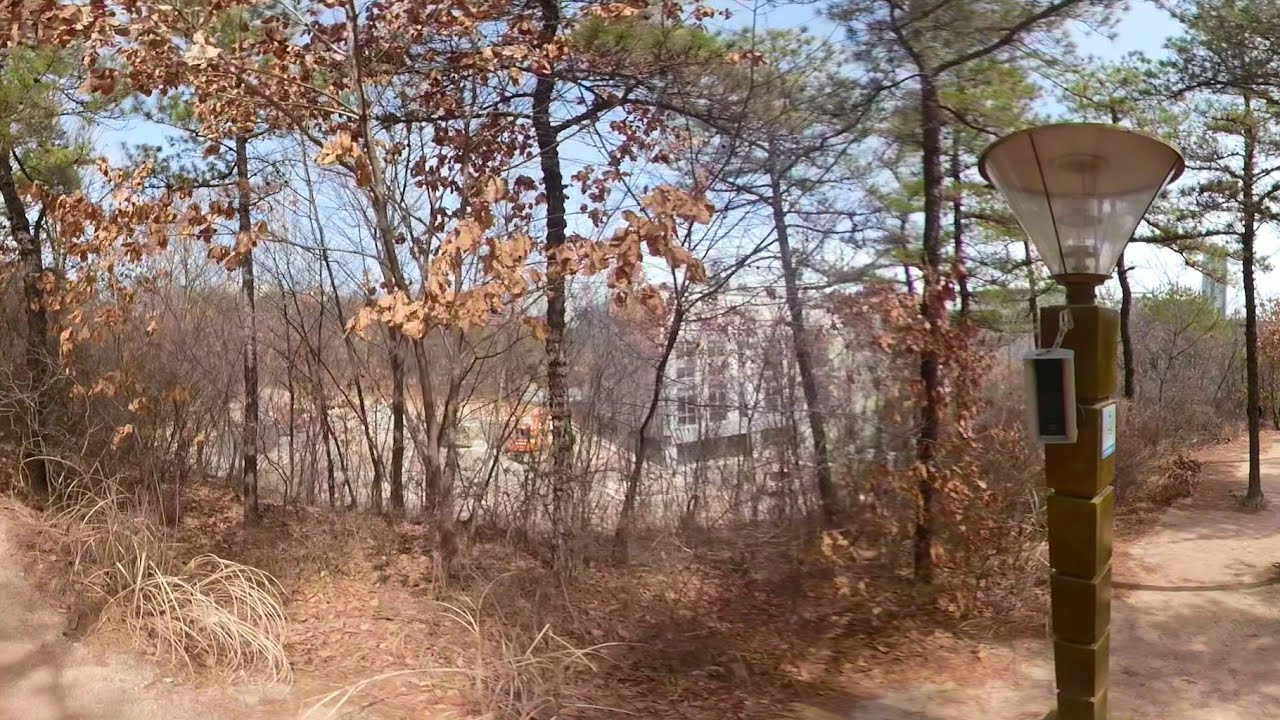The image has a picturesque, almost painting-like quality, showcasing an outdoor scene with a mixture of trees and greenery. In the foreground, there is an interesting metal lamppost with a cylinder-shaped light hanging from it, possibly functioning as an entrance marker or feature for a pathway or park area. This lamppost seems to have some sort of keypad, suggesting it could be part of an entry system, maybe to a large estate or residential property. The scene features a diverse array of trees, some still lush with green leaves, particularly to the left and top center, while others have dried brown leaves, indicating it could be autumn. The landscape spreads out with ample shrubs and muted hues, contributing to the tranquil ambiance. In the background, a large building partially obscured by the trees hints at a substantial property or perhaps a large business or institutional building, creating a strong focal point amidst the natural setting. This setting gives the impression of a spacious estate or perhaps a suburban walking path with rich and varied natural elements, all captured in a wide-angle shot that slightly distorts the scene, providing an expansive view of this tranquil outdoor space.